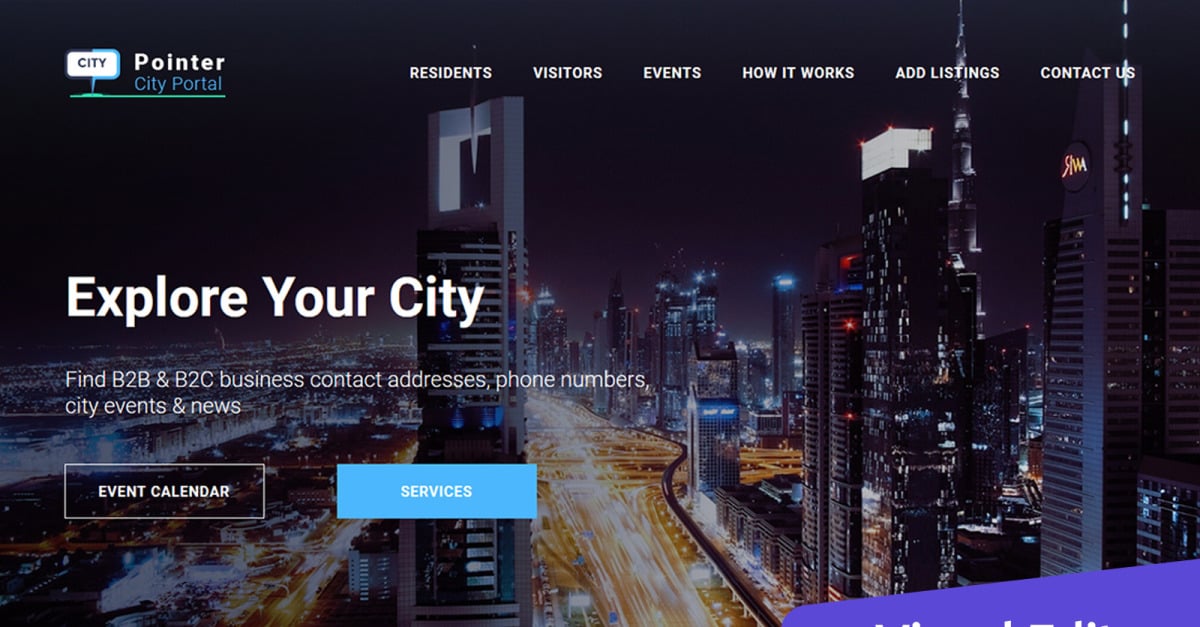### Detailed Caption for Image:

The top-left corner of the image features the text "Pointer City Portal." The word "Pointer" is displayed in white, while "City Portal" appears in blue. To the left side, there's a white and blue pointer, underlined in green, labeled "City" beneath the "Pointer City Portal." 

Located at the top-right corner are several white tabs arranged horizontally across the page, starting from the left with the following labels: "Resident," "Residents," "Visitors," "Events," "Outworks," "Ad Listing," and "Contact Us."

Central on the left side of the image is the phrase "Explore Your City," followed by an informational text: "Find B2B and B2C business contact addresses, phone numbers, city events, and news."

At the bottom of the image are two distinct buttons. The left button reads "Event Calendar" in white, with no shading, while the right button says "Services" in blue.

The background of the image depicts a vibrant cityscape at night, filled with city lights, traffic lights, and moving cars. The streetlights and vehicle lights create yellow trails on roads and bridges. 

Prominently positioned slightly left of center is a building with an illuminated white "M" on its top. To the right side of the image, another building has a glowing yellow logo with the letters "RWA" clearly visible on its top right.

This detailed view captures the dynamic and intricate design of the Pointer City Portal interface alongside a bustling urban landscape.